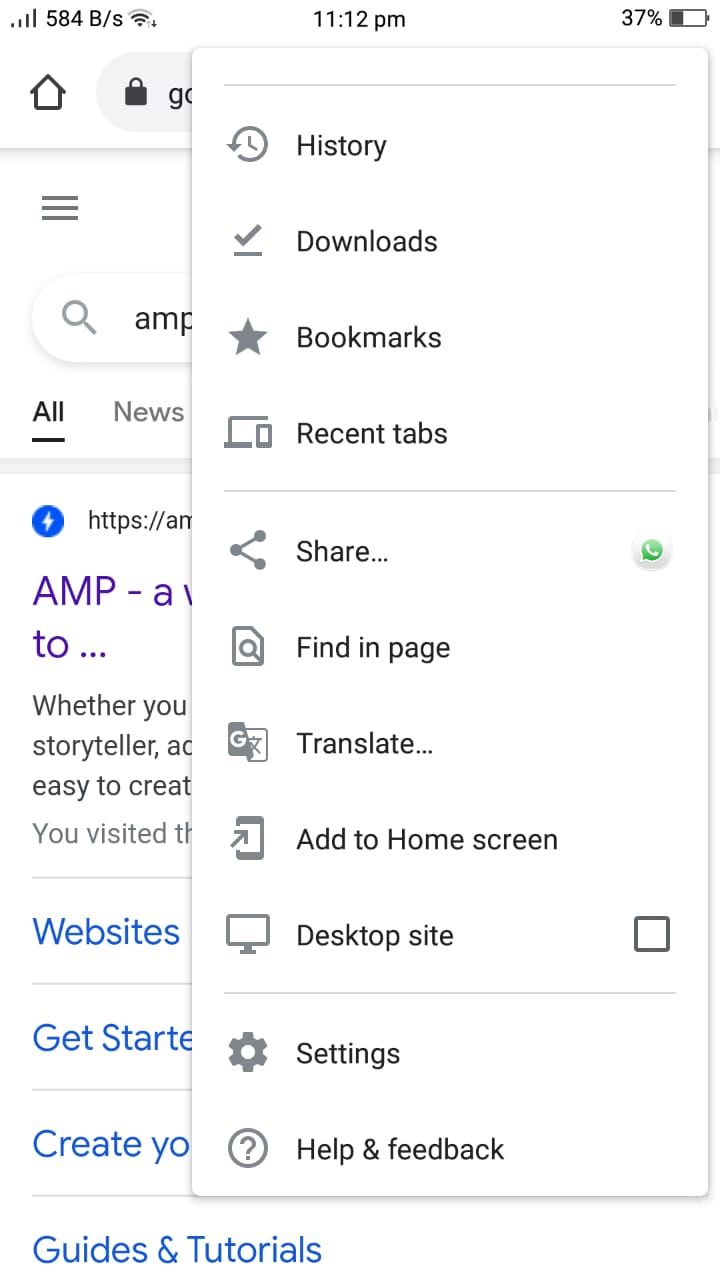The image is a screenshot from a smartphone with a white background. At the top left, the time displayed is 11:12 p.m., while the battery indicator at the top right shows a charge of 37%. The central focus of the image is a vertical list of items in a gray font. Each item is accompanied by a corresponding icon on its left. The list includes:

- History
- Downloads
- Bookmarks (with a gray star icon)
- Recent Tabs
- Share
- Find in Page
- Translate
- Add to Home Screen
- Desktop Site
- Settings
- Help and Feedback (with a gray circle around a question mark icon)

The list appears as an overlay on top of the background, which shows a partially visible Google search results page. The search term at the top of the background is "AMP," but the content is mostly obscured by the overlay menu.